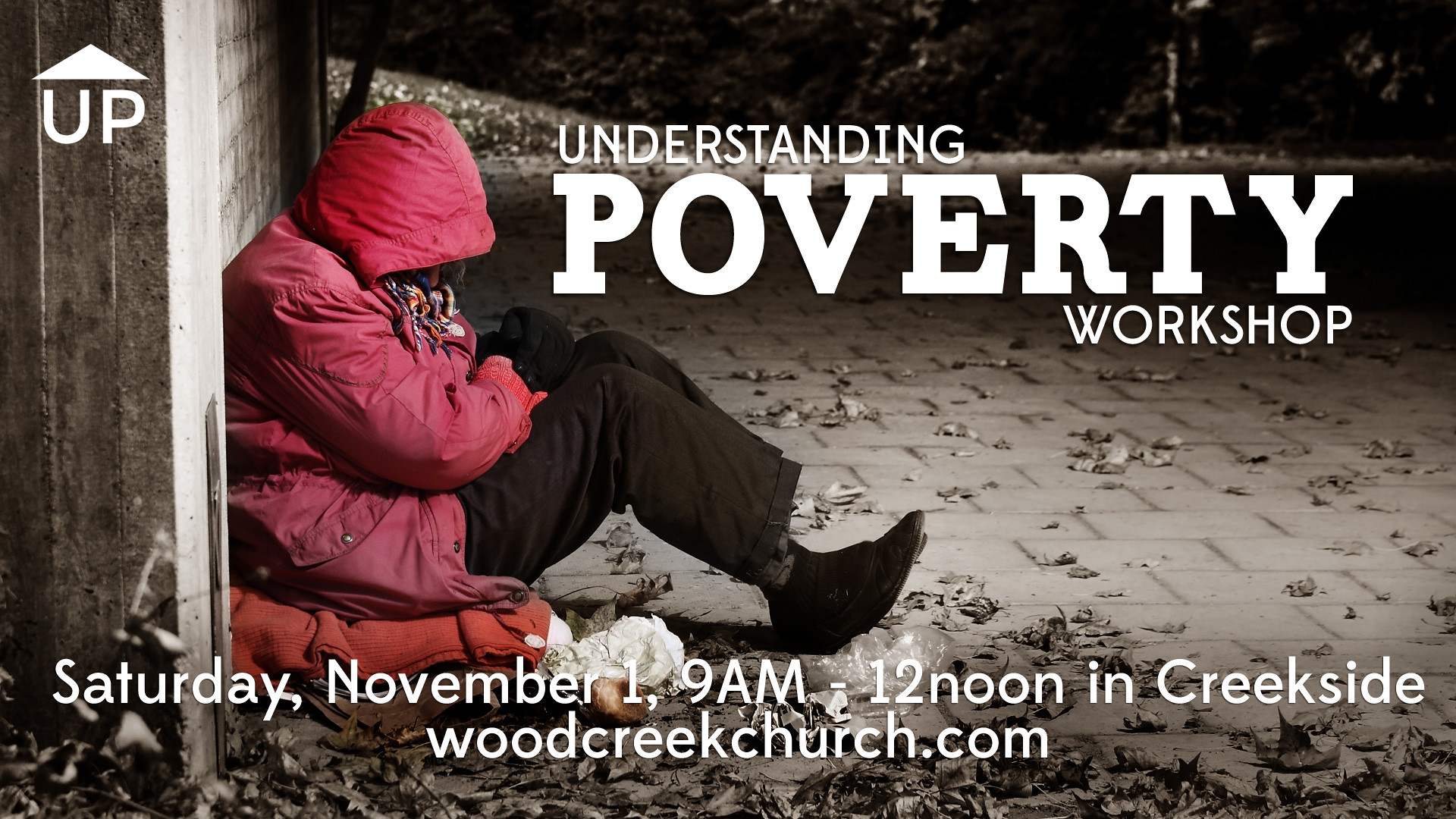The image is a poster depicting a homeless person sitting on the ground outdoors at night, illuminated by overhead lighting. The individual, seen from a side profile, is hunched over and wrapped in a piece of clothing that is spread on the ground beneath them. They are wearing a red puffy coat with the hood up, obscuring their face, along with long black pants and black shoes. They are seated amidst dirt and old dead leaves, leaning against what appears to be either a tree or a wall. The poster includes white text, prominently featuring "Understanding Poverty Workshop" with the word "poverty" in large letters. Below the image, additional text provides details: "Saturday, November 1, 9 a.m. to 12 noon in Creekside, woodcreekchurch.com."